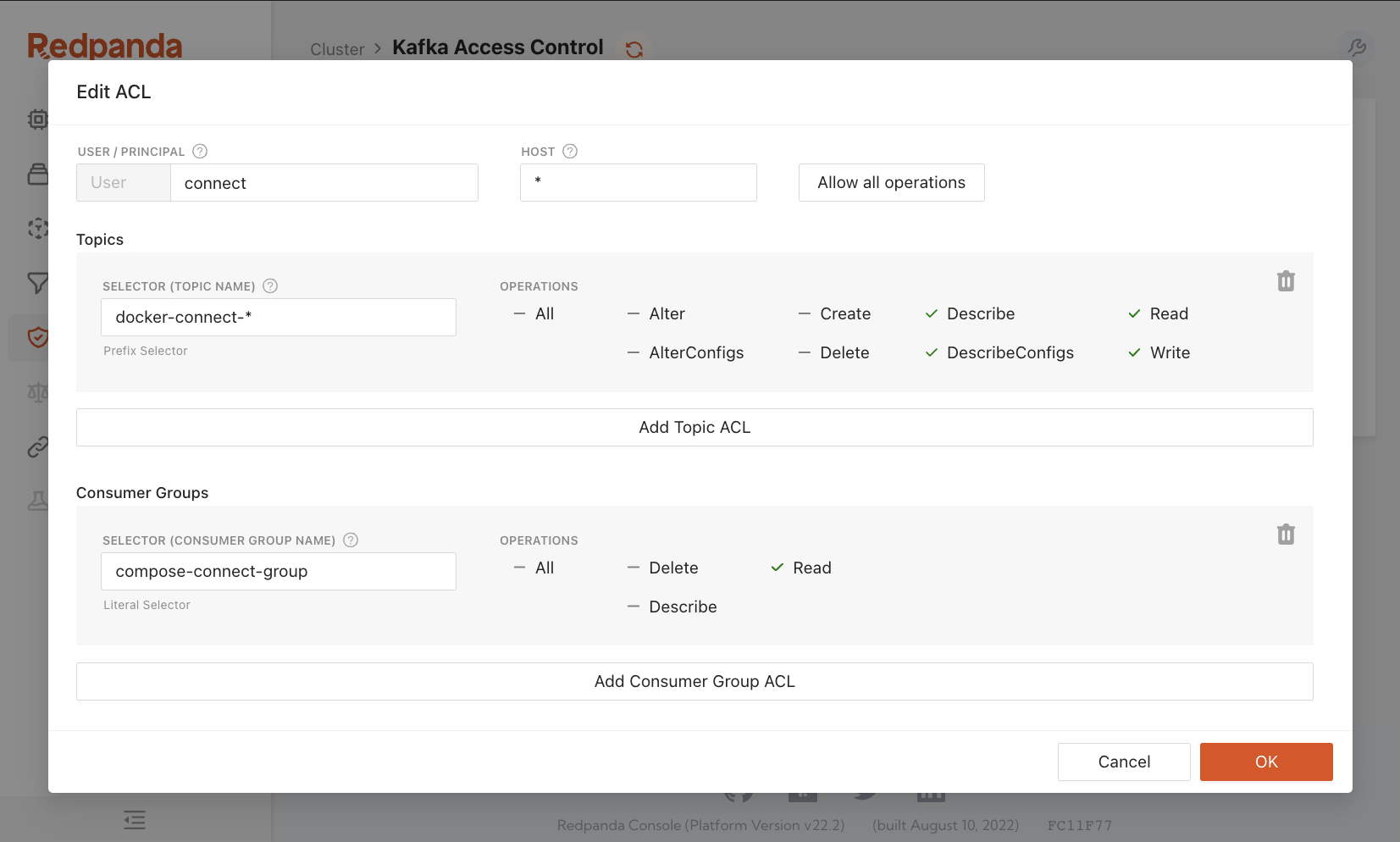The screenshot captures the "Edit ACL" window from a computer application interface. In the foreground, a user with the username "userconnect" is currently connected. The interface displays a single host, denoted by an asterisk (*) under the host bar. The topics section lists "selector/docker/connect/*," encompassing operations including "All," "Alter," "Alter Configs," "Create," "Delete," "Describe," "Describe Configs," "Read," and "Write." Below this, there is an option to add additional topic ACLs.

Further down, the consumer groups section shows a group named "compose/connect-group." The operations available for this group also include "All," "Delete," "Describe," and "Read." Users can add additional consumer group ACLs as well.

At the bottom of the window, two buttons are visible: an orange box labeled "OK" in white font, and another box labeled "Cancel." Flanking these buttons are two grey-colored trash bin icons, presumably for deleting entries.